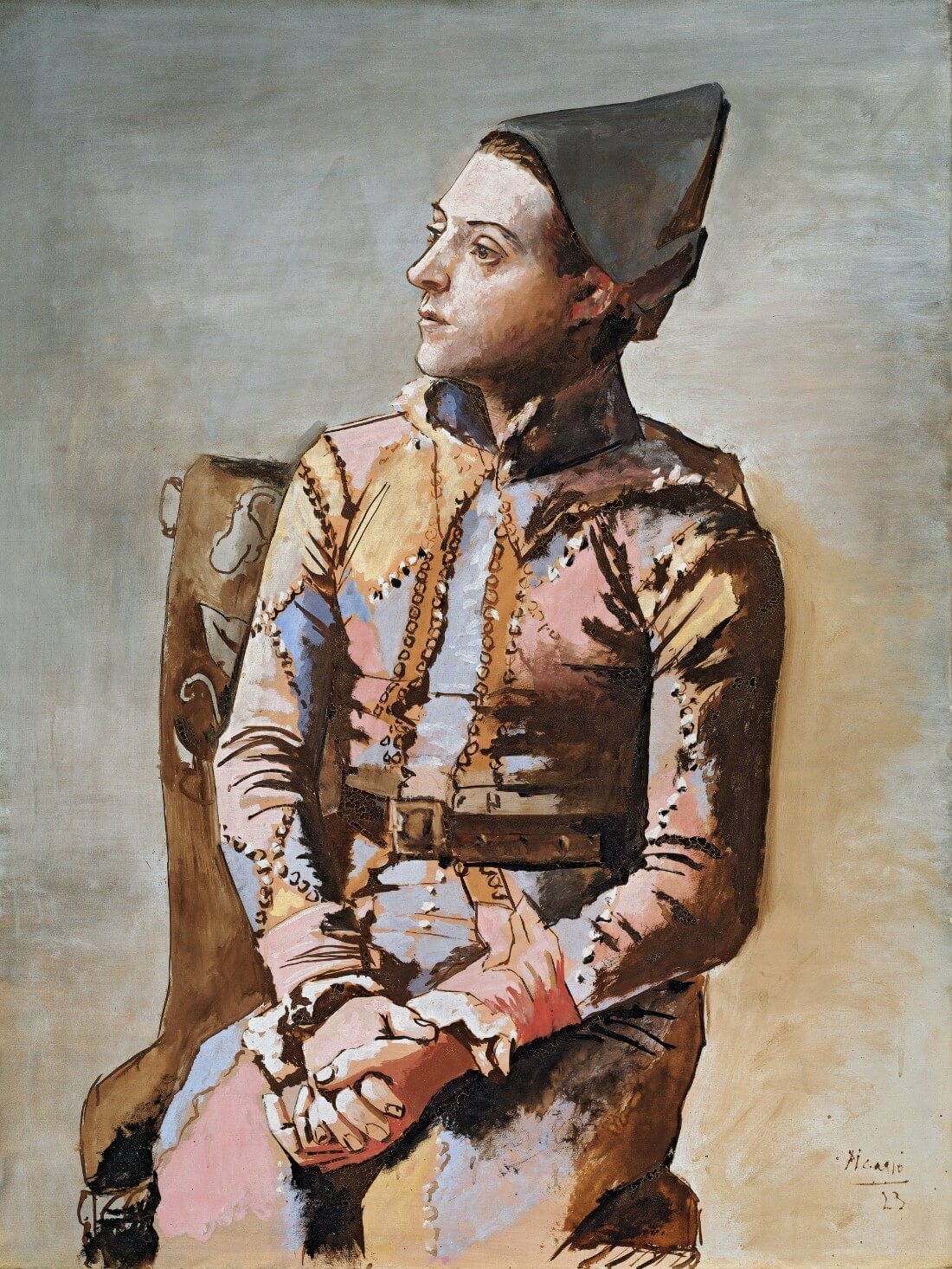This is a painting attributed to Picasso, as indicated by the small signature in the bottom right corner. The artwork features a man sitting in a wooden chair, gazing off to the left with a neutral expression. The background exhibits a gradient from gray at the top to a sepia-toned brown or cream at the bottom. The man, who appears to be a white figure from a bygone era, sports a pointed hat that is either brownish-gray or black and has short, closely cropped brown hair. His facial features include a notably triangular and sharp nose. He is dressed in a striking, multi-colored jacket and pant ensemble adorned with diamond-shaped patterns in hues of pink, blue, brown, yellow, and orange, complemented by a large collar and several buttons. A brown belt cinches his waist, and his hands are clasped together in his lap. The painting, executed in watercolor and ink or pencil, showcases muted colors and a modest level of detail.